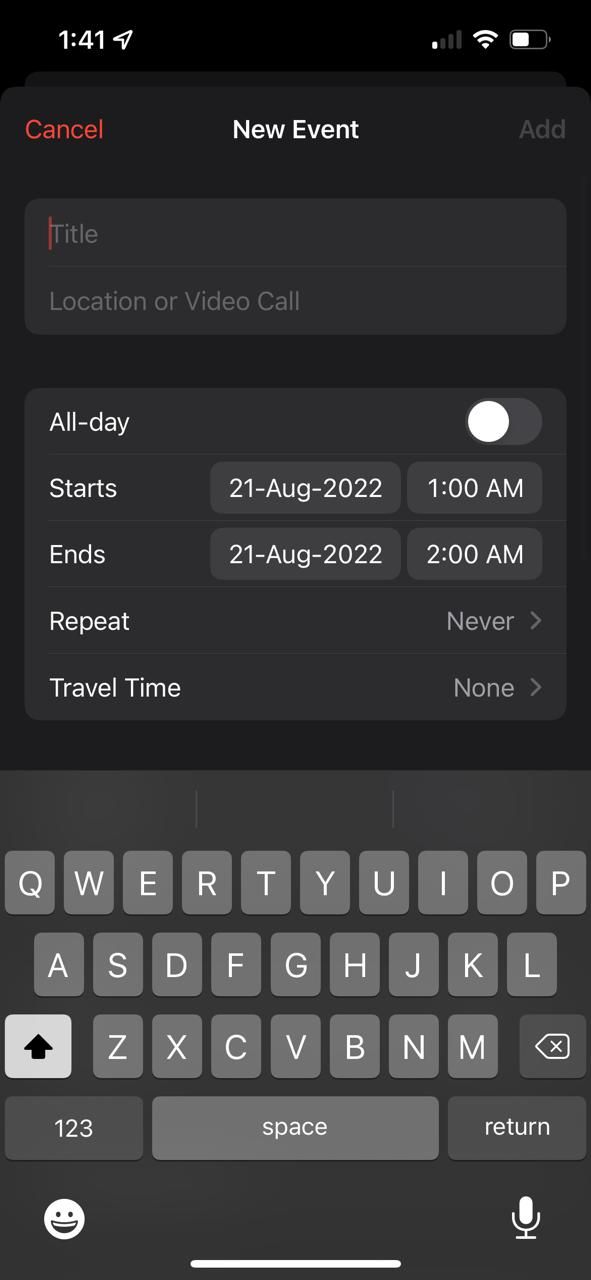The screenshot captures the process of setting up a new event on a smartphone calendar application. At the very top of the image, the black status bar displays the time "1:41" in white, along with several icons indicating one bar of cellular signal, full Wi-Fi connectivity, and a battery at half capacity. Below the status bar, a dark gray window occupies the screen's central area, featuring the title "New Event" prominently in the center. On the left side of this window, a red "Cancel" option allows the user to discard the event setup, while on the right side, a gray "Add" option enables the user to save the event.

The interface includes two primary input fields: one for the title of the event and another for specifying the location or setting up a video call. Beneath these fields, the event scheduling options are displayed. An 'All-day' toggle is positioned to the right of the 'All-day' label, set to the off position. The 'Starts' field shows the date and time "21 Aug 2022 1:00 AM" and is followed by the 'Ends' field, indicating "21 Aug 2022 2:00 AM." Additional options include 'Repeat', set to "Never," and 'Travel Time', set to "None."

At the bottom of the screen is a basic QWERTY keyboard featuring three rows of light gray keys with white letters. The space bar and the return key are similarly styled. A white emoji icon is visible in the bottom left corner, while a white microphone icon is positioned in the bottom right of the keyboard, all set against a light gray background.